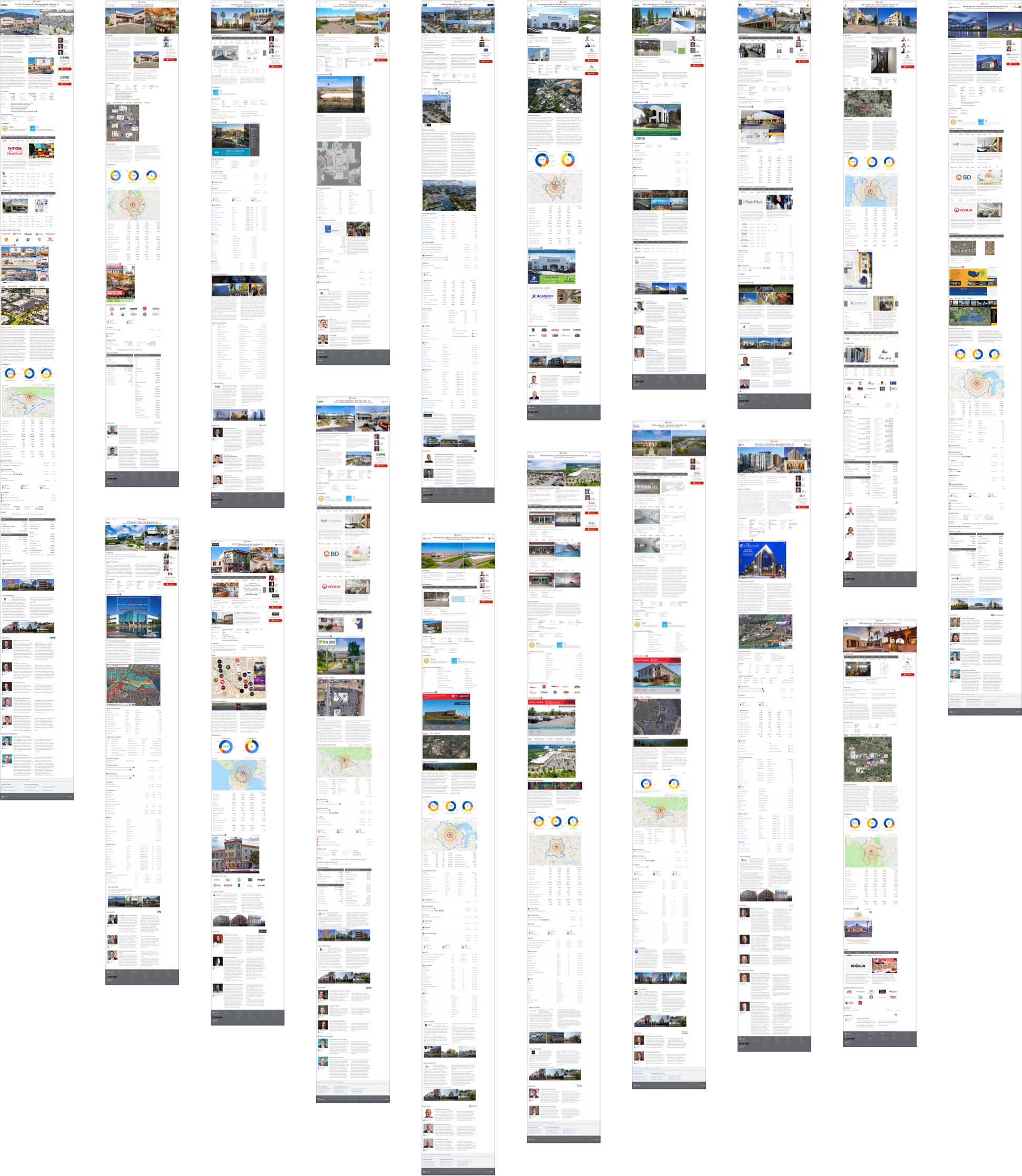This detailed caption describes the image:

A white background hosts a meticulously arranged collage of elongated, rectangular boxes that resemble web pages or threads, all presented in portrait orientation. The arrangement consists of ten columns that alternate in height and configuration, creating a cascading effect from the edges toward the center. The outermost columns feature single, extremely tall web pages, each stretching approximately six to nine times their width. Adjacent to these are columns containing two stacked rectangular boxes, separated by white space, appearing slightly longer as they progress inward. This pattern continues until the central columns, which exhibit the longest pages of all. The lack of defined borders and the consistent white backdrop emphasize the vertical orientation and varying lengths of each page or thread, suggesting a sense of intentional design despite the unclear purpose. The image overall gives the impression of overlapping or extended web pages, meticulously aligned to form a cohesive and visually intriguing presentation.